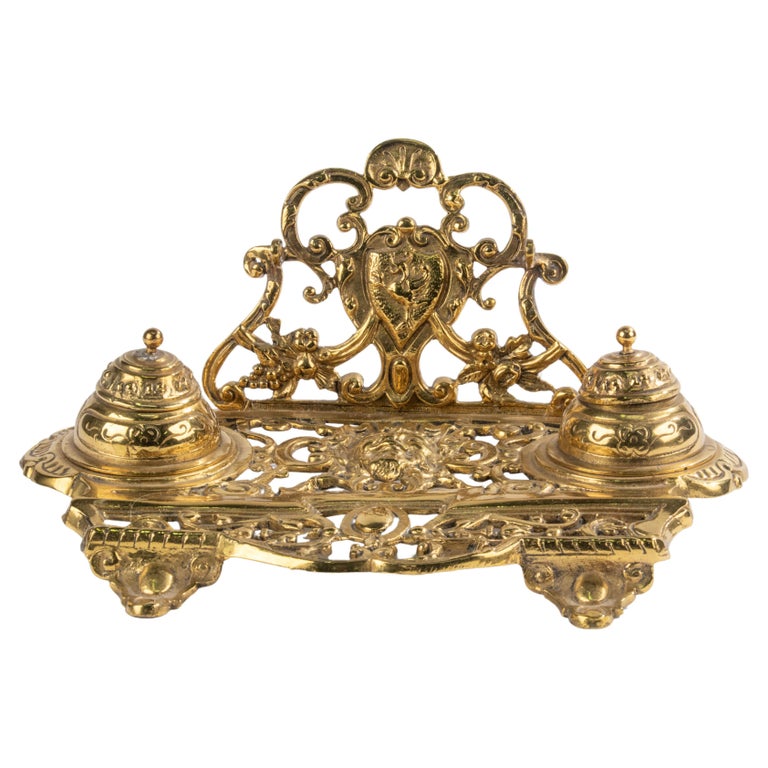This image depicts an ornate, vintage decorative item, likely gold or gold-plated, which appears to have originated from the early 1900s or earlier. The structure is reminiscent of a small table or stand, with intricately carved, slightly rounded feet that it rests on. Symmetrical on both sides, the main feature of the base is a rectangular tray-like platform, which might serve a functional purpose such as storage.

Elevating from the back of this tray is a vertical structure adorned with an elaborate crisscross looping pattern of gold. This vertical extension culminates in an emblem resembling the face of an owl, positioned centrally at the top. The owl design includes curled edges and an oval-shaped face, giving it a distinctive appearance. Interspersed within this looping design are open spaces that provide visibility through to the background.

Flanking the main platform, on either side, are two bell-shaped objects, reminiscent of hand-pushed bells, similar to those used for ringing at a hotel reception. These appear functional and can be lifted off the tray, hinting at a possible dual-purpose design where the tray stores items underneath these bell-like covers.

In addition to the owl figure, the piece boasts multiple motifs and intricate patterns, including floral and fruit shapes, giving it a rich, ceremonial aesthetic. The central backing also features a badge-like emblem with a pair of wings atop, complemented by detailed brass lines that add to the ornamentation. The lower section of the structure, slightly bell-shaped, is further enhanced by curls and round sections, contributing to the overall vintage and ornate appeal of the decoration.

This detailed and multifaceted item showcases an intersection of functionality and artistic craftsmanship, embodying both aesthetic beauty and potential historic significance.